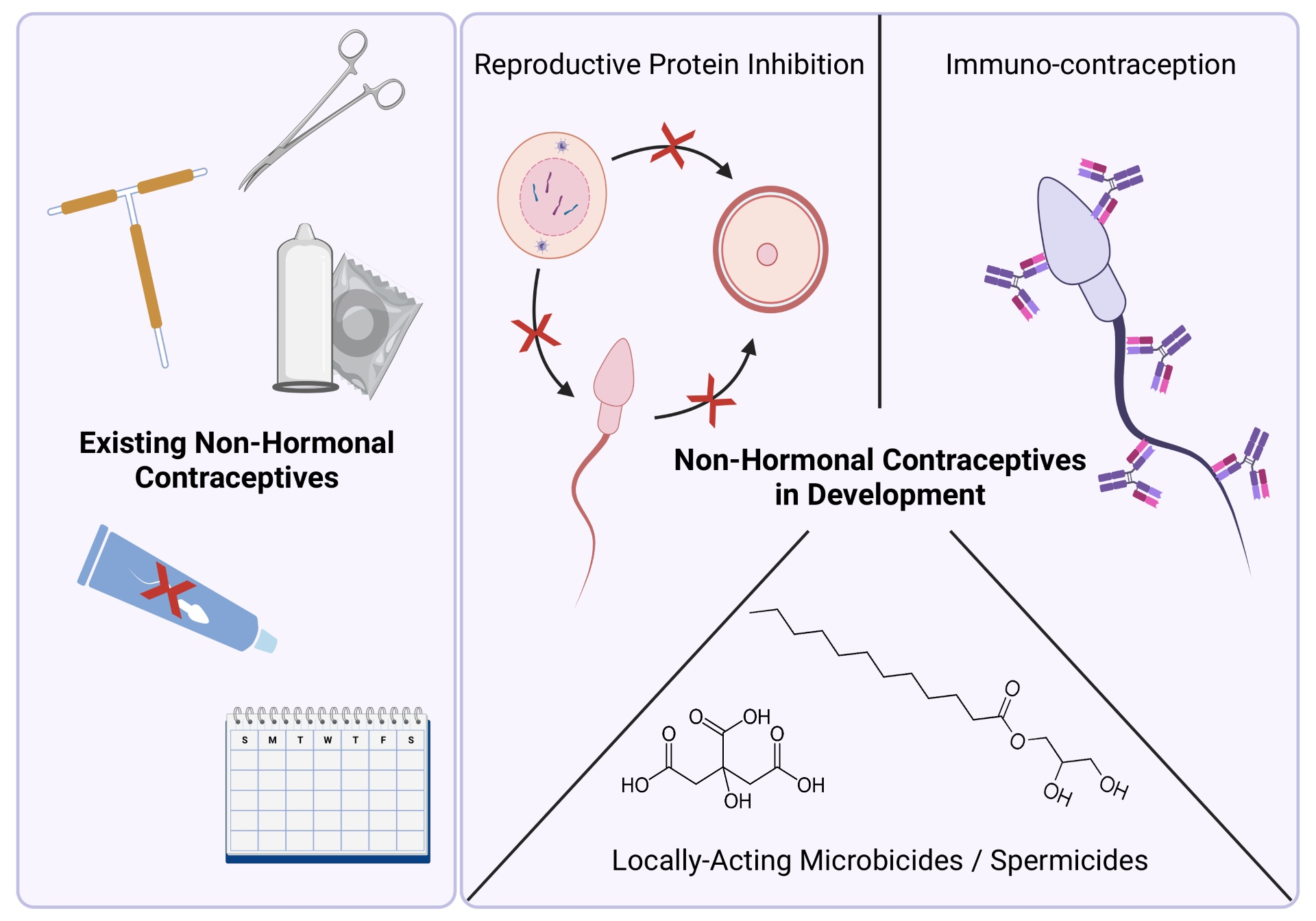The image is a detailed infographic on contraception, particularly focusing on non-hormonal methods. The background is a pale purple or pink, giving it a medical and informative appearance. The infographic is divided into sections that explain various types of contraceptives.

The first section, labeled "Existing Non-Hormonal Contraceptives," includes visual elements such as scissors (indicating vasectomy), a toothpaste-like tube (possibly representing spermicidal jelly), condoms, and a calendar for fertility planning.

The second section is labeled "Reproductive Protein Inhibition." It features a diagram of the reproductive system with arrows marked with X's, indicating the inhibition points of the reproductive proteins.

The third section, "Immunocontraception," displays a diagram of a sperm surrounded by different colored lines, likely representing antibodies or immunological barriers. Additionally, this section highlights "Non-Hormonal Contraceptives in Development," illustrating concepts like locally acting microbicides and spermicides with a diagram resembling a chemical formula.

Overall, the infographic comprehensively details various existing and developmental non-hormonal contraceptives, using clear visual aids and descriptions to convey the information.